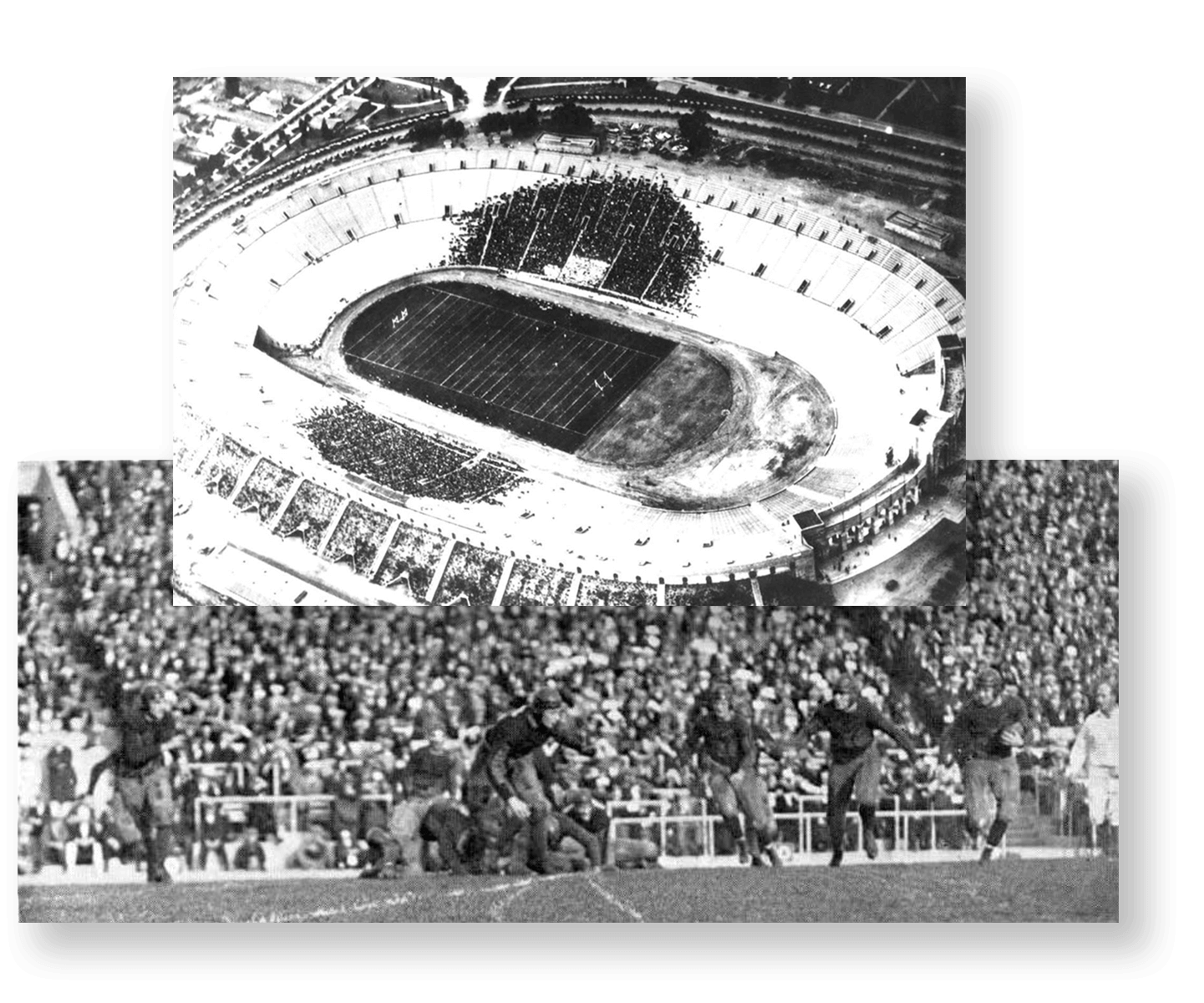This vintage, black-and-white composite photo features two distinct images of a historic football game at the Los Angeles Coliseum. The top image is an impressive aerial view of the snow-covered stadium, surrounded by roads and trees, giving an overview of the seating arrangement with scattered spectators. The bottom image captures a moment during an early 20th-century football game, likely from the 1930s to 1950s, showcasing players in old-fashioned uniforms and leather helmets on the field. The stadium seats are filled with a large, attentive crowd, highlighting the event's significance. The detailed vintage setting provides a nostalgic glimpse into the early days of American football.